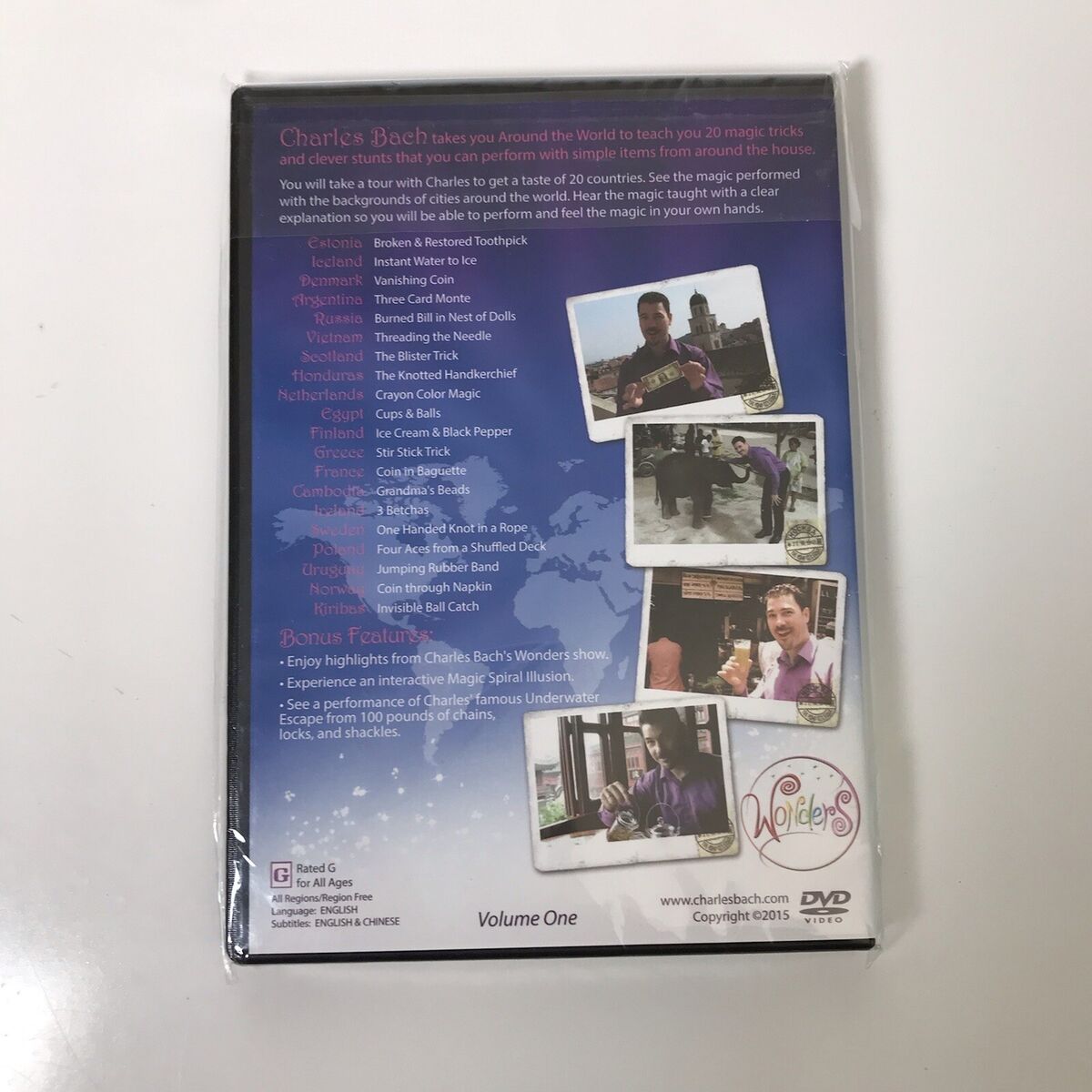The back cover of this DVD, encased in a black cellophane-wrapped case, invites you to join Charles Bach as he takes you around the world to teach 20 magic tricks and clever stunts using simple household items. The top of the cover features text highlighting this adventure. On the right side, four sequential photographs showcase Charles in various vibrant settings: first, he is holding up a dollar bill while standing before a European temple; second, he is petting a baby elephant while wearing a blue shirt and gray pants; third, he sports a white jacket and holds a glass of a beverage; finally, he is seated at a table, pouring something into a cup. The background of the cover is gray with a black rim at the top, offset by a blue area resembling a map and a white section with water droplet graphics in the left corner. The DVD title, "Wonders," is displayed in a colorful, fancy script within a red circle. Additional text details Charles's magical tour across 20 countries, including Estonia, Iceland, Denmark, Argentina, and others, with highlights from his show, bonus features, and an underwater escape performance. The DVD is marked as Volume 1 and is rated G for all ages, released in 2015.